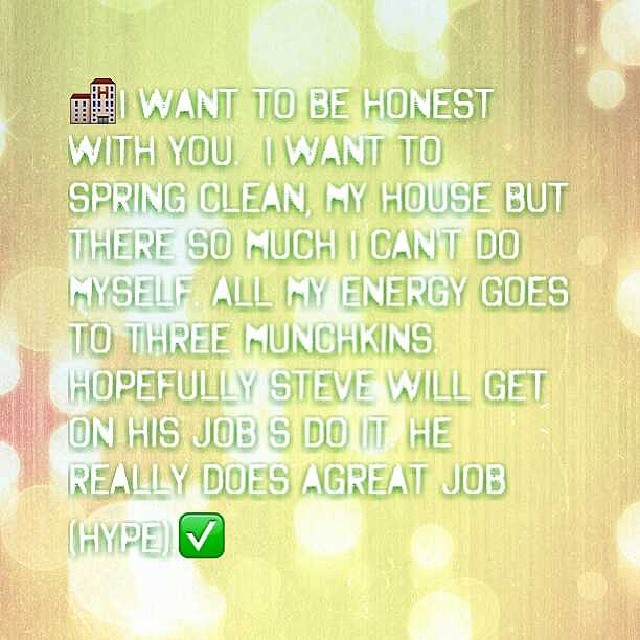This square digital poster features a soothing pastel background that transitions from light green to warm reds, oranges, and yellows, with faint vertical lines adding a subtle texture. Scattered throughout the background are delicate white spheres of light, reminiscent of glowing orbs. 

Centrally located, a paragraph in all capital white letters with a green border stands out. The text appears in a bold, 1980s computer font and opens with a hospital emoji and closes with a green checkmark emoji. The message reads: "I want to be honest with you. I want to spring clean my house, but there's so much I can't do myself; all my energy goes to three munchkins. Hopefully, Steve will get on his job. Do it. He really does a great job. Hi."

This poster, likely resembling an Instagram or Twitter post, includes a concise, informal note that reflects a mix of personal confession and hopeful encouragement, complete with an erratic yet genuine tone.